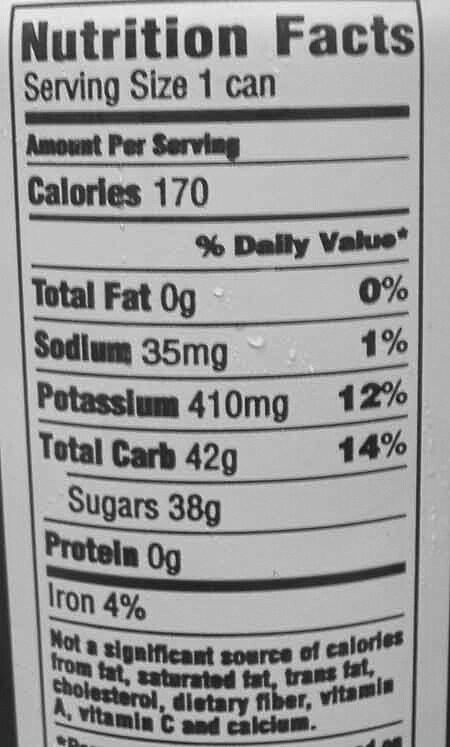This image displays a nutrition facts label commonly found on food packaging. The label features black text on a white background and provides comprehensive nutritional information for the contents of one can. The details include:

- Serving Size: One can
- Calories: 170 
- Percent Daily Values:
  - Total Fat: 0%
  - Sodium: 35 mg
  - Potassium: 410 mg (12%)
  - Total Carbohydrates: 42 g (14%)
  - Sugars: 38 g
  - Protein: 0 g
  - Iron: 4%

Additionally, the label notes that the product is not a significant source of calories from fat, saturated fat, trans fat, cholesterol, dietary fiber, and vitamin D.